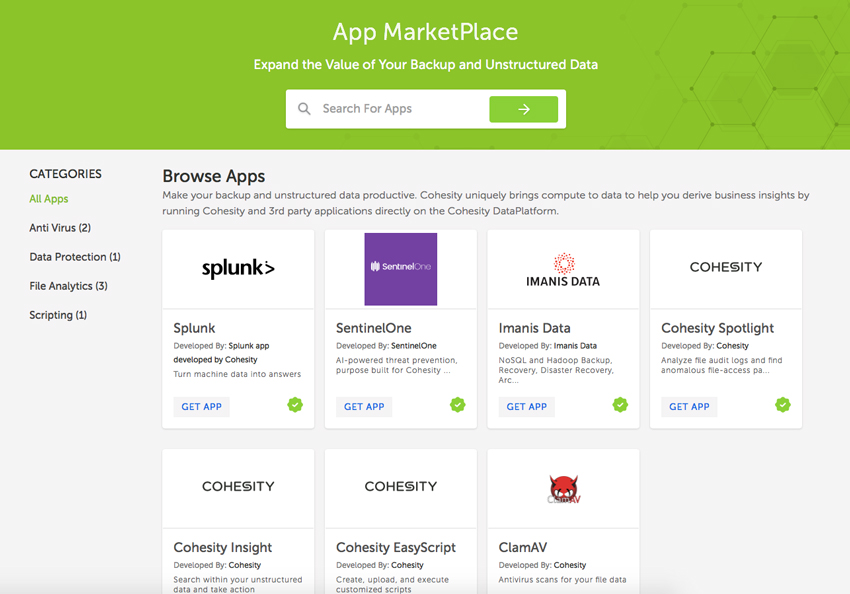Screen capture from the App Marketplace website highlighting features of Cohesity's data management platform. The webpage header reads "Expand the Value of Your Backup and Unstructured Data" and includes a search bar for locating apps. Below the header, there are filter options to browse all categories or select specific types of apps such as antivirus, data protection, file analytics, and scripting.

The section on application offerings emphasizes how Cohesity enables businesses to maximize their data's utility by integrating compute capabilities and running Cohesity and third-party applications directly on the Cohesity data platform. Listed applications include Splunk for data analysis, SentinelOne for cybersecurity, Imanis Data for complex data management, Cohesity Spotlight for operational insights, Cohesity Insight for data visibility, Cohesity EasyScript for simplified scripting, and Clam AV for antivirus protection.

The capture succinctly illustrates how users can leverage various specialized apps to transform their backup and unstructured data into actionable business insights, thereby enhancing productivity and security within the Cohesity ecosystem.